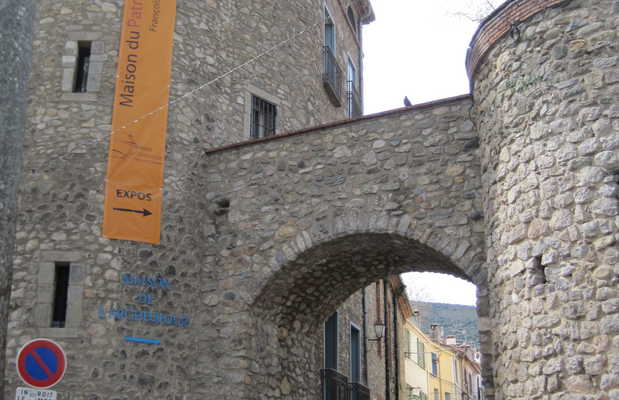The photograph captures a detailed view of a stone masonry building, likely a historic castle, illuminated by daylight under a light blue sky. The structure features a prominent round tower on the left side, connected by an arched stone bridge to another rounded tower on the right. The focal building is intricately constructed with old-school windows and spans at least two stories. Below the stone archway, additional buildings are visible; the nearest is yellow, and others in the distance vary in color, including a reddish-brown hue. An eye-catching bright orange banner on the left side of the building bears the partial French text "Maison du P.A.T.R." and the word "Expos" in black font with a right-pointing arrow. The architectural details and connected structures speak to a rich historical context, juxtaposed with modern signage.